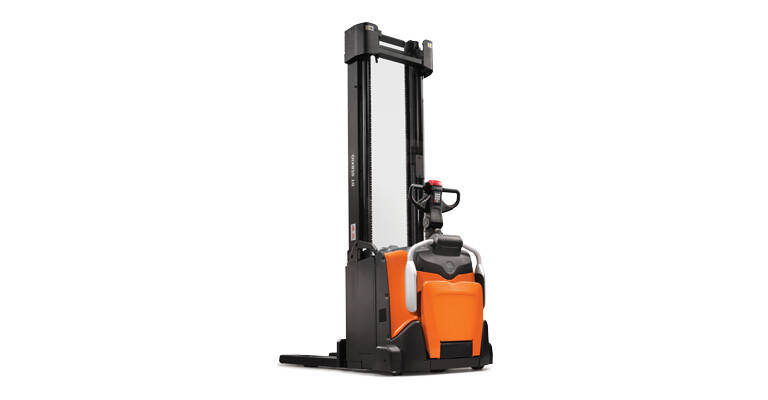The image displays a centrally positioned electric stacker truck against a solid white background. The truck features a tall, rectangular lift at the back with a black frame and a silver, metallic center. The front part of the machine is predominantly orange, comprising a seat and steering wheel with a red button on top. Below the steering wheel, there is a distinctive silver arch over a black surface. The base of the truck houses the black fork mechanism. The equipment appears to be designed for operator use, incorporating handles and various control tools. The entire truck, showcasing colors of black, orange, silver, and gray, nearly fills the image, suggesting it could be promotional material for industrial equipment, possibly from a retailer like Home Depot. The image contains no text.